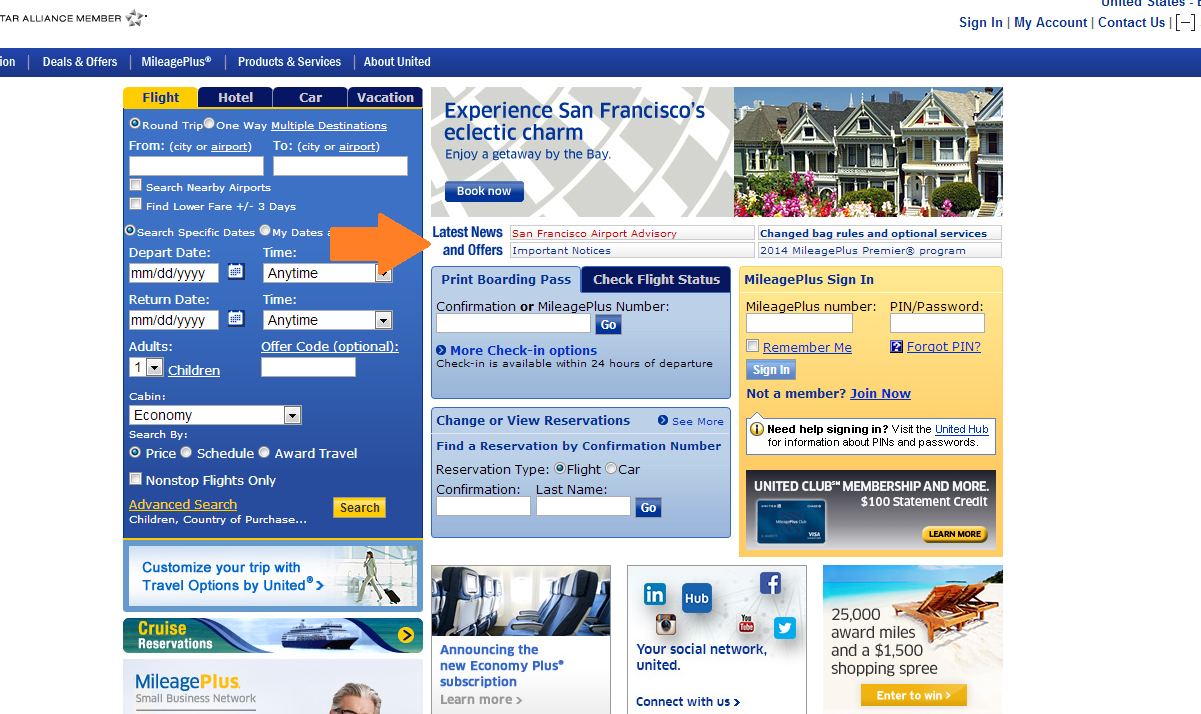The image is a detailed screenshot of a computer display showcasing a travel website, likely belonging to United Airlines. At the top left corner, partially cut off, is the logo indicating "TAR Alliance member." A prominent blue navigation bar spans the top of the screen with various menu options including "Deals and Offers," "Mileage Plus," "Products and Services," and "About United."

Beneath this blue bar, there is a slightly narrower rectangle segmented into various interactive fields. In the upper left of this rectangle, the title "Flight" is highlighted in yellow, and adjacent options such as "Hotel," "Car," and "Vacation" are also visible. This section includes input fields for vital travel details: departure date, return date, destination, origin, and travel class (economy, first class, etc.). At the bottom right of this box, a yellow button labeled "Search" allows users to initiate a search for flights.

Under this primary rectangle, there are smaller boxes offering additional functionalities, such as customizing trips with various travel options provided by United Airlines. Prominently placed in the center is a module promoting travel to San Francisco, with the headline "Experience San Francisco's Eclectic Charm, Enjoy Getaway by the Bay." A small blue "Book Now" button is positioned at the lower left of this promotional section.

Additional service boxes are scattered across the screen, allowing users to print their boarding passes, and change reservations. There is also a "MileagePlus Sign-Up" box highlighted in yellow on the right center. In the upper right corner of the screen, there is a small image depicting a row of iconic, narrow houses characteristic of San Francisco, enhancing the city's allure as a destination.